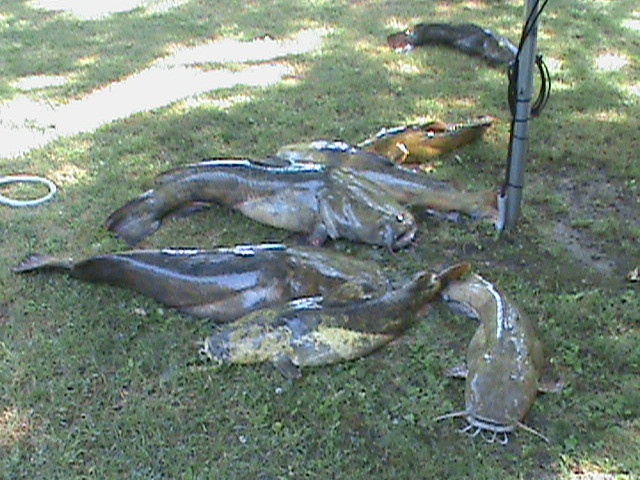The photograph captures an outdoor scene on a bright, sunny day. The ground, which is grassy with a sandy undertone, is largely covered in shadows, but sunlight filters through the trees behind the camera, casting a warm glow. Featured prominently are at least six large, freshly caught catfish, still glistening with water. Their slimy bodies suggest they are recently out of the water, with one fish, in particular, showing its distinctive whiskers toward the camera. Positioned off to the right is a metal pole with black cables wound around it, and a white rope is visible in the bottom right corner of the image. The catfish vary in size, possibly weighing five to six pounds each, and one is notably a golden color. They are scattered haphazardly on the ground, further emphasizing the fresh, rustic nature of the scene.